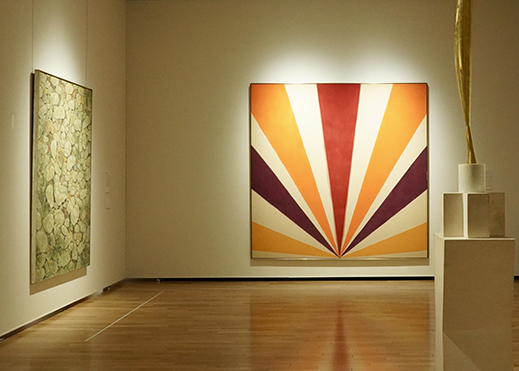The image captures the interior of an art gallery with brown hardwood flooring that appears lacquered and polished. The walls, painted in a gray-beige or cream color, frame a corner where two large square paintings are displayed. The painting on the left wall is an abstract piece with mixed hues of green, white, and gray, featuring indistinct shapes that evoke a sense of a populated lily pad. The painting on the far wall is more detailed; it features seven broad rays radiating from the bottom center against a light beige backdrop. The central ray is red, flanked by orange, dark purple, and a pair of yellow, creating an alternating color pattern. In front of this painting, there is a conspicuous golden rod sculpture. The gallery uses a tape line on the floor to denote a safe viewing distance from the artworks, offering a modern alternative to traditional velvet ropes.